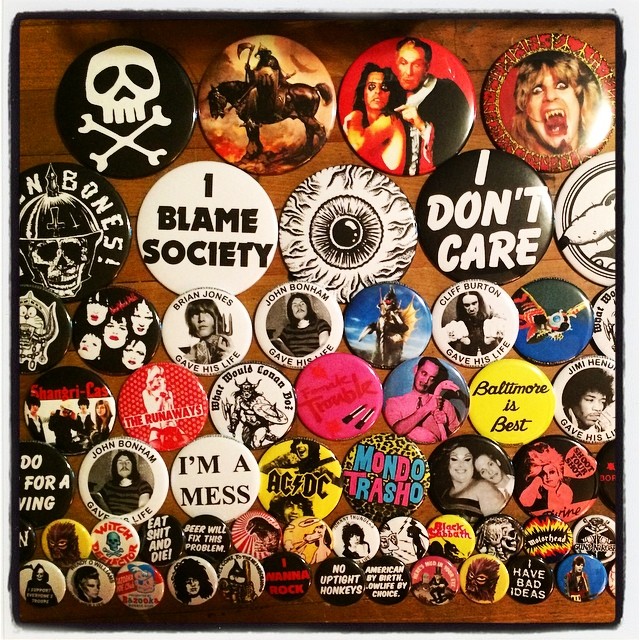This square graphic features a grungy, sketchy border and appears to be a wooden surface with a dark, burnt reddish-brown hue. It's adorned with numerous button pins that vary significantly in size, with the largest ones positioned at the top and gradually decreasing in size towards the bottom. Notable buttons include a black pin with a white skull and crossbones, an image of Ozzy Osbourne with fangs, and several with bold text such as "I blame society," "I don't care," "I'm a mess," and "Cliff Burton gave his life." Other notable pins feature an eyeball design, a skeletal face, and references to iconic bands like AC/DC and The Runaways. Additional buttons display quirky and rebellious messages, such as "Baltimore is best," "What would Conan do," "Mondo Trasho," "No uptight honkies," "Shoot your shot," "Eat shit and die," "Beer will fix this problem," "Black Sabbath," "Metal head," "I have bad ideas," "American by birth, low life by choice," and "I wanna rock." The collection exudes a punk and rebellious spirit, reflecting a diverse range of cultural and musical references.